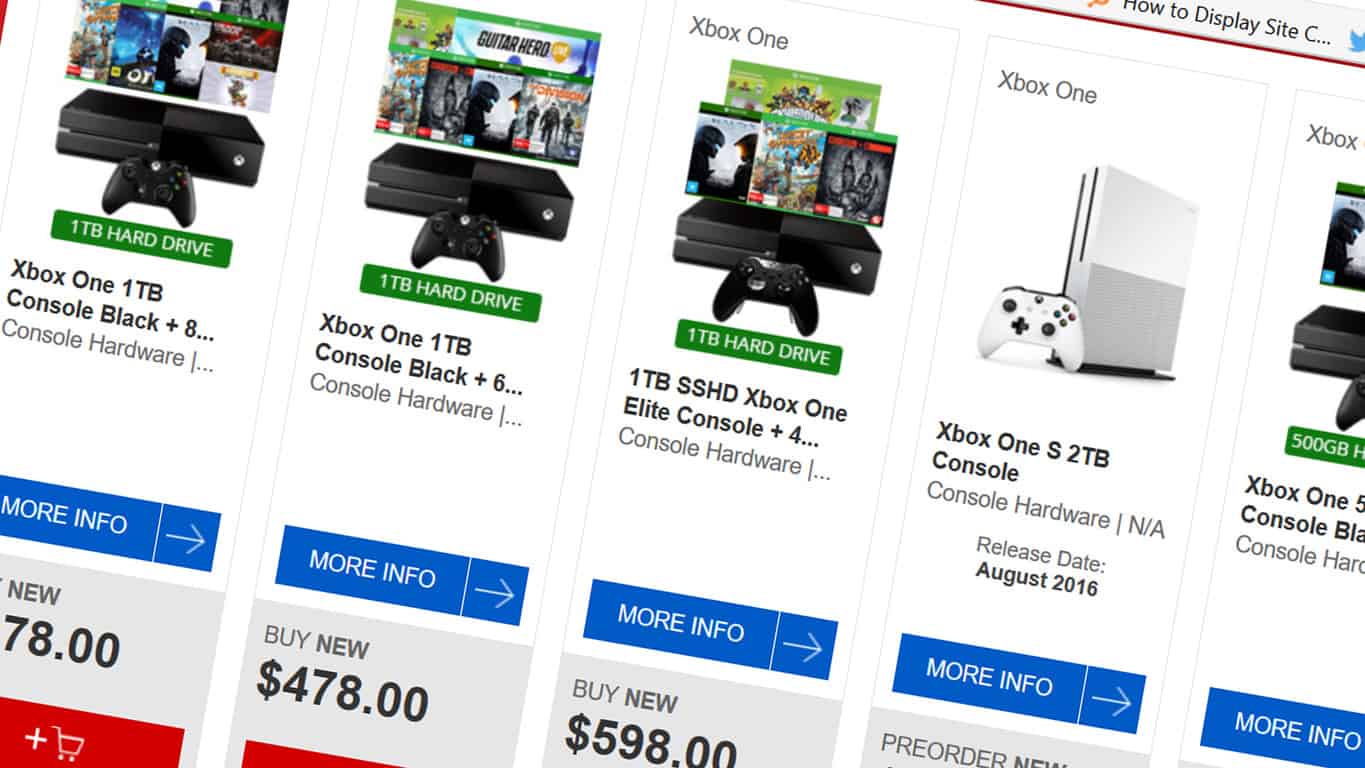The image is a slightly tilted screenshot showcasing various Xbox One console models available for purchase. In the upper left corner, there's a tab indicating a display option setting, emphasizing that this is indeed a screenshot. From left to right, the first item listed is an Xbox One 1TB black console alongside unspecified console hardware, with the price partly obscured, showing only $78. The second item is an Xbox One 1TB console black with accompanying hardware priced at $478. Next is a 1TB SSHD Xbox One Elite console paired with additional hardware, priced at $598. These first three consoles are black with matching black game controllers. The fourth item deviates from the pattern; it is an Xbox One S 2TB console, oriented vertically and colored in white and gray, with a release date set for August 2016. Unfortunately, the price for this model is not visible. All five items in the image are different models of the Xbox One console, highlighting their various specifications and configurations.